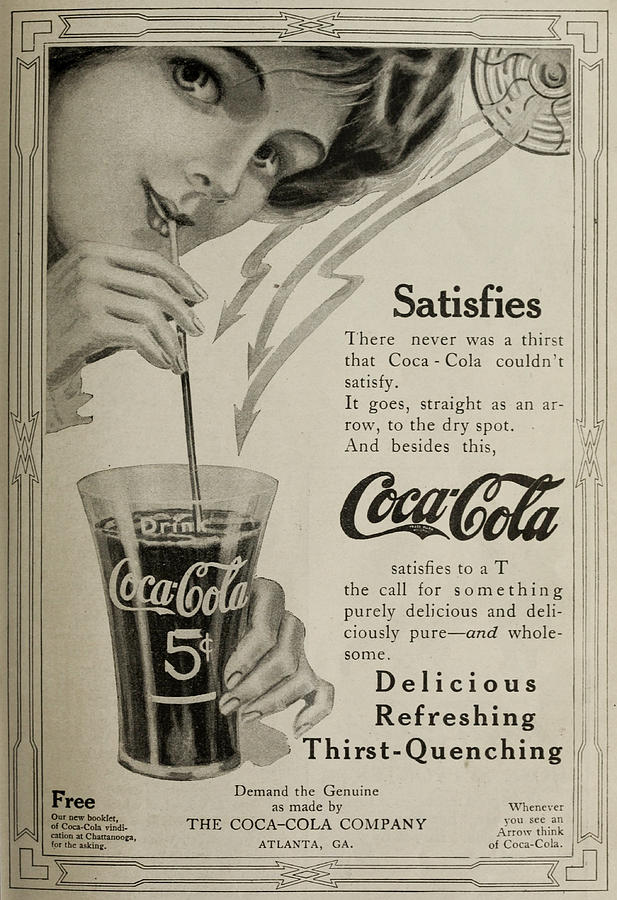This vintage black-and-white Coca-Cola advertisement, possibly from the 1920s, features a hand-drawn illustration of a stylish, doe-eyed woman in the upper left corner. The woman, reminiscent of the Victorian Gibson Girl with the shape of her hair, tilts her head into the image and gently smiles while holding a straw to her lips with her right hand. She appears quite elegant, with a hint of makeup and a fancy sleeve cuff visible. Her left hand is disconnected from her body, shown holding a glass labeled "Coca-Cola" and "five cents" in white text. 

To the upper right, the image includes a metal fan depicted with motion waves or arrows blowing air towards the glass, adding a dynamic element to the design. The ad is bordered with an ornate frame that evokes styles akin to Art Deco or Art Nouveau, enhancing its vintage charm. 

Prominent text on the right side of the image reads, "Satisfies. There never was a thirst that Coca-Cola couldn't satisfy. It goes straight as an arrow to the dry spot. And besides this, Coca-Cola satisfies to a T. The call for something purely delicious and deliciously pure and wholesome. Delicious, refreshing, thirst-quenching." Additional text near the bottom left offers a free Coca-Cola booklet. In the center, it states, "Demand the genuine as made by the Coca-Cola Company, Atlanta, Georgia," and the lower right advises, "Whenever, wherever you see an arrow, think of Coca-Cola." The old paper tint adds to the nostalgic feel of this elaborate and striking advertisement.